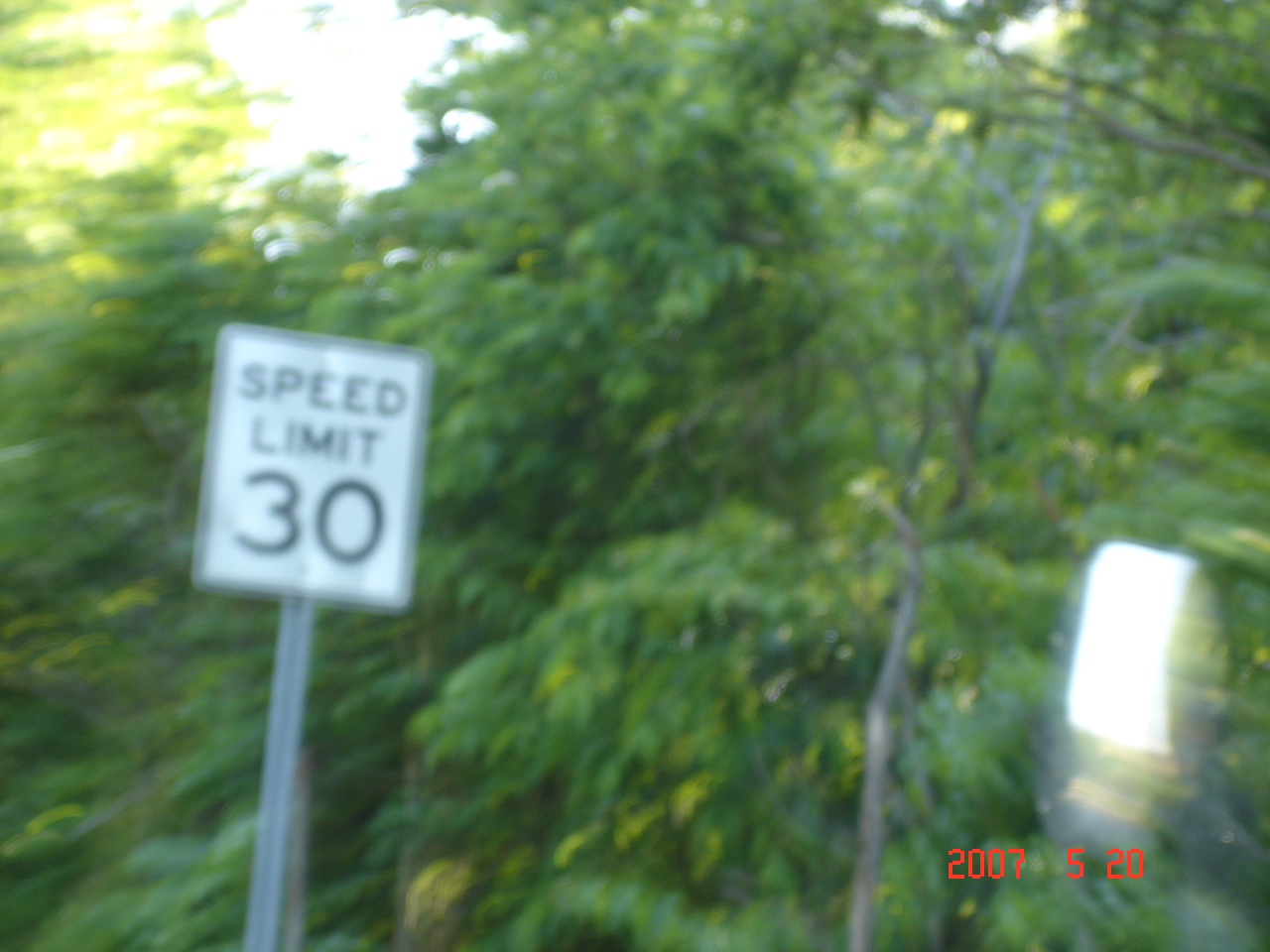In this photograph, the primary focus is a street sign indicating a speed limit of 30 mph. The sign, featuring bold black text and a black border on a white rectangular background, is mounted on a metal pole situated on the left side of the image. Surrounding the sign is a dense array of foliage, with various trees, leaves, and branches filling the background, creating a lush, green backdrop. Adding a subtle timestamp to the scene, the bottom right corner of the image includes a red date stamp reading "2007 520," with a slight glare visible above the date due to the way the picture was taken.